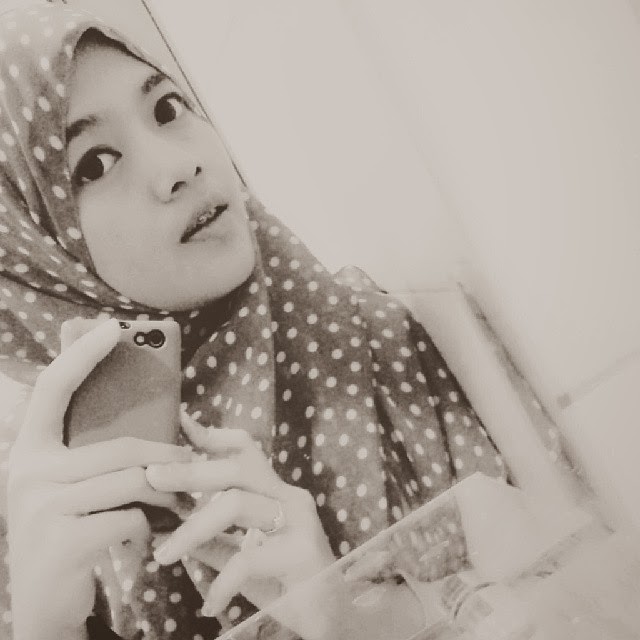This black and white photograph captures a teenage girl taking a selfie in front of a mirror. She wears a polka-dotted hijab that covers her hair and drapes down in front of her chest. The angle of the image places her head in the top left corner, and you can tell she is holding a cell phone, likely an older model iPhone, in both hands—her right hand positioned in front of her right shoulder and her left hand supporting the phone from the bottom. She gazes forward and slightly to the right with dark eyes, her mouth half open, revealing her braces. A ring adorns the second to last finger on her left hand. Due to the high contrast and monochromatic nature of the photo, the exact colors are indiscernible, leaving only the strong visual impression of her determined yet slightly surprised expression. In the background, a plastic ledge is visible across the bottom right of the image, adding a subtle context to her surroundings which are otherwise ambiguous.